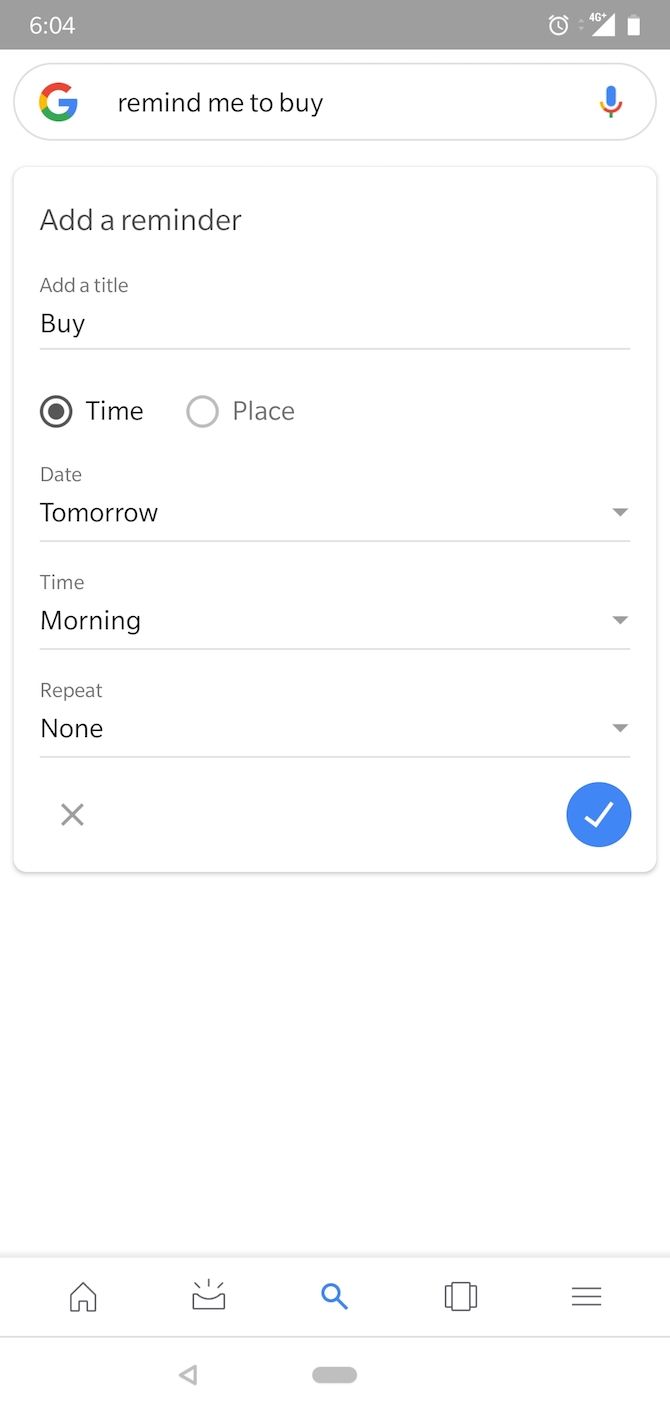A smartphone screenshot showcases a reminder setup screen within the Google Assistant or Google Search interface. The device, potentially an iPhone or Android, displays the current time as 6:04 (unclear if AM or PM). The status bar indicates a 4G connection with a fully charged battery. The search bar at the top displays the user’s input, "remind me to buy," initiating the reminder creation process. Below the search bar, the interface offers fields for further details: the reminder title is simply "buy." The user opts to set the reminder for "tomorrow morning" with no repetition, as indicated by the "none" option under the repeat settings. A prominent blue checkmark button located at the bottom right corner enables the user to confirm and save the reminder upon completing their input.